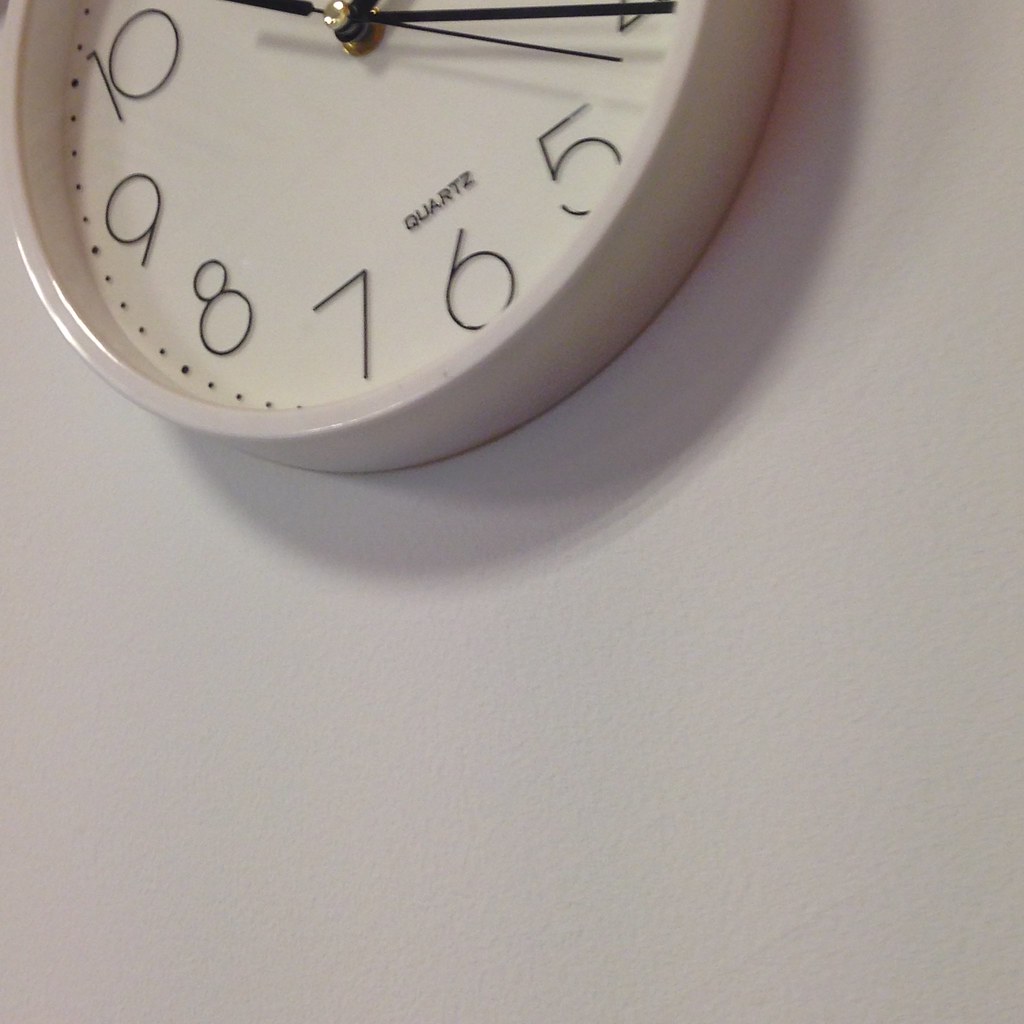This photograph captures a close-up, off-center view of a wall clock taken from a slightly low angle, revealing approximately three-quarters of the clock face. The clock features a minimalist design—a completely white face contrasted by bold black hands and numbers. Only the numbers 4 through 10 are visible, with the time showing around 11:20. The word "Quartz" is also prominently displayed near the center of the clock. Minute markers, represented by small dots, encircle the perimeter of the clock face. The background is an eggshell white wall, which appears to be somewhat worn, with a few visible marks. The absence of any people or additional text in the photo makes it challenging to determine the exact setting, though it could plausibly be a domestic space, such as a kitchen or living room.